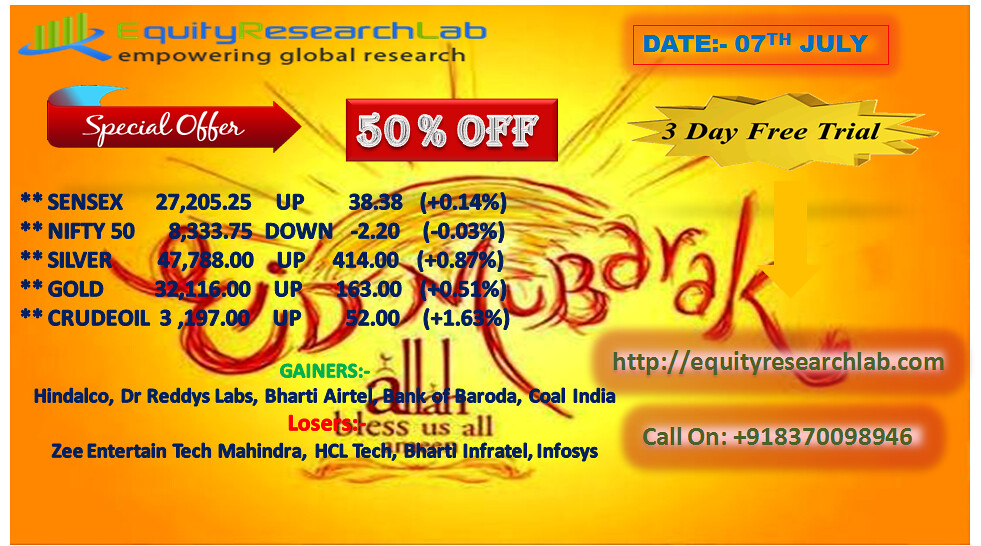The image is a vibrant, computer-generated advertisement predominantly in shades of yellow and orange. At the very top, in blue letters with green initials, it says "Equity Research Lab" followed by "Empowering Global Research" in black text. On the upper right, within an orange outline, it mentions the date, "7th July." Below that, there is a section bordered in yellow stating "3-Day Free Trial," alongside a prominent red banner declaring a "Special Offer" of "50% Off."

On the left side, a flat, microscope-like graphic contains four green cylindrical shapes extending from it. The image features various financial details, including a list of commodities and stock indexes with their trading values, such as Sensex, which is up by 38.38 points, Nifty 50, Gold, Silver, and Crude Oil. It also highlights the "Gainers" and "Losers" of the market. At the bottom right, the website "http://equityresearchlab.com" and a phone number are provided for further contact.